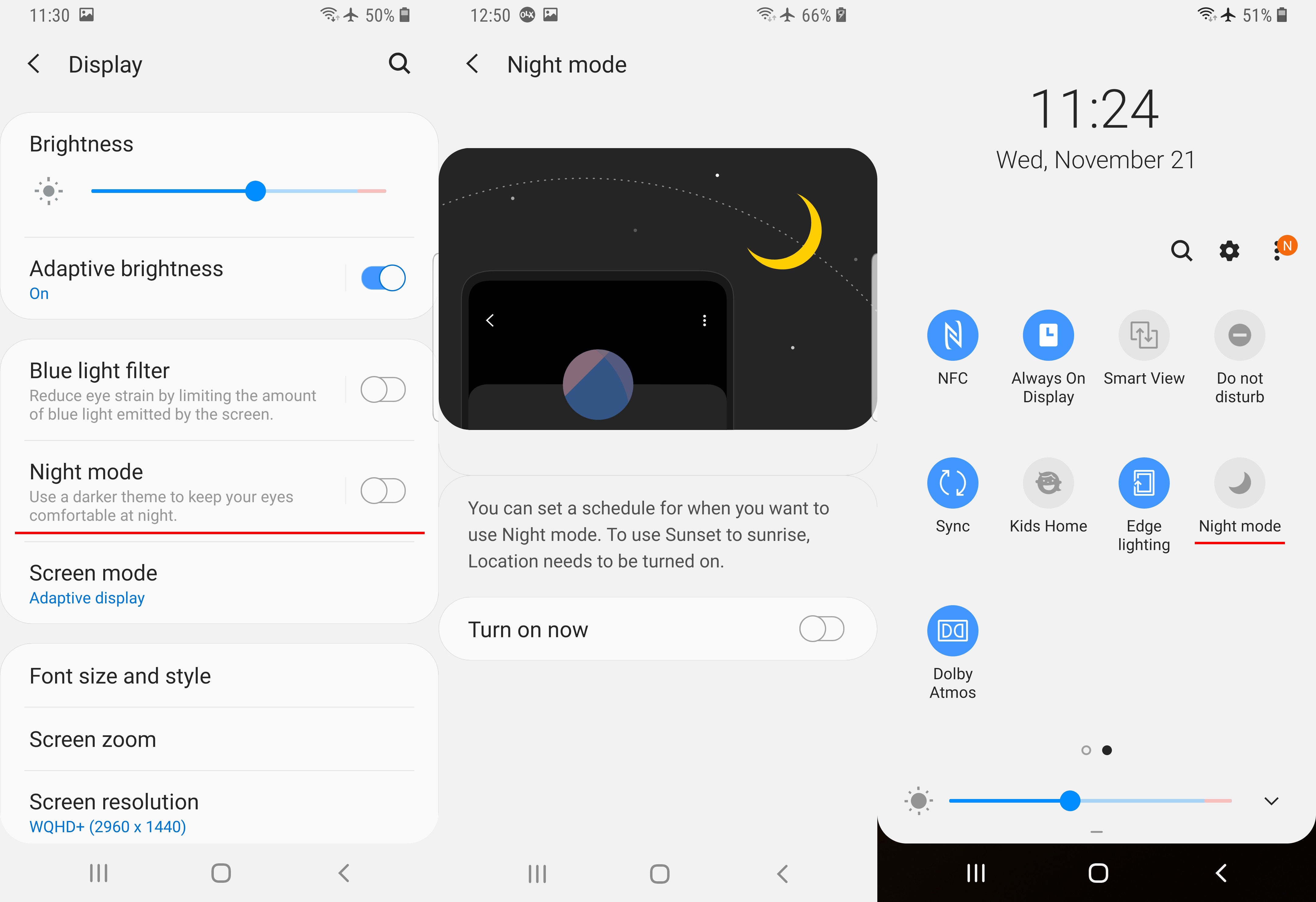The image showcases three distinct screens from a smartphone, detailed as follows:

1. **Left Screen - Display Settings:**
   - A comprehensive overview of display settings, featuring a brightness slider, an adaptive brightness switch, and a blue light filter toggle set to off.
   - Night mode is also turned off, and options for screen mode adjustments are present.
   - Additional controls include font size and style, screen zoom, and screen resolution.

2. **Middle Screen - Night Mode Settings:**
   - This screen displays the settings for Night Mode, illustrated with an image of a night sky and moon.
   - Users can set a schedule for Night Mode, such as from sunset to sunrise, which requires location services to be turned on.
   - There is a checkbox and a switch to enable Night Mode immediately.

3. **Right Screen - Quick Settings:**
   - The quick settings menu is displayed, showing the current date and time: Wednesday, November 21st, 11:24.
   - Below, we see several toggles for features like NFC, Always On Display, Smart View, Do Not Disturb, Sync, Kids Home, Edge Lighting, Night Mode, and Dolby Atmos.
   - NFC, Always On Display, Sync, Edge Lighting, and Dolby Atmos are activated, while the rest are turned off.
   - All three screens show the current time in the top left corner, except the rightmost screen, which does not.
   - The top right corner of all screens shows battery status and connectivity icons for Wi-Fi and cellular service.